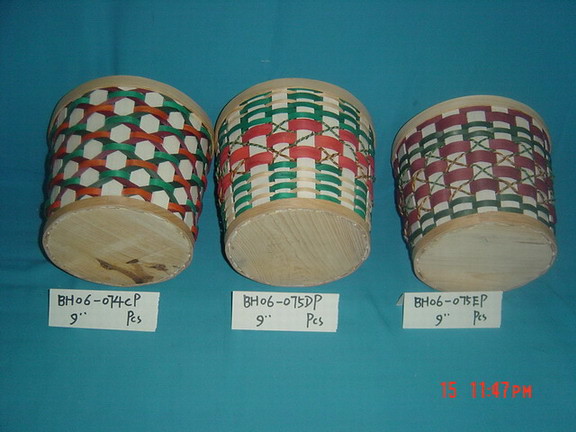This photograph showcases three small, cylindrical woven baskets displayed against a tealish blue cloth background. Each basket is positioned on its side, revealing their circular bottom and distinct woven patterns. The leftmost basket features a light brown weave with hexagonal shapes and colorful stripes in green, orange, and pink. Beneath this basket, a white sheet of paper with numerical annotations is visible, suggesting dimensions or model identification, including the symbol for inches. The central basket is similarly light brown with green, white, and red stripes, its decorated middle section featuring an undulating swirl of red boxes. The rightmost basket, in a light wooden brown hue, displays crisscross red, green, and white stripes. An orange timestamp, "151147pm," is situated at the bottom right of the photo. Each basket has a corresponding white tag that likely contains further details or measurements, enhancing their presentation as labeled artifacts.